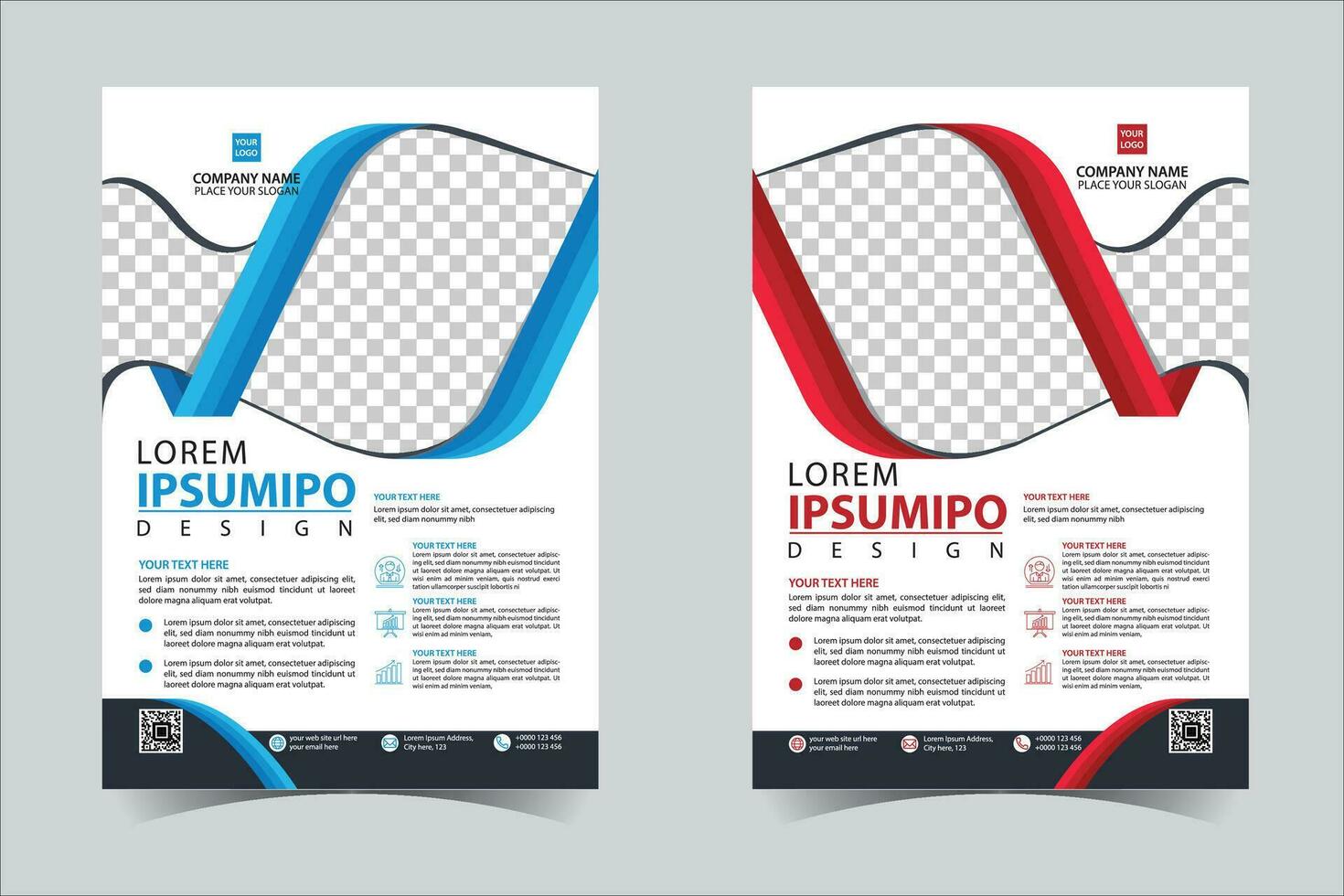The image is a promotional template likely intended for advertising products or services, which can be customized by various companies. Featuring a neutral gray background, the template presents two almost identical flyer designs side by side, differing only in color scheme. 

On the left, the flyer showcases a blue ribbon that partially encloses a designated area for a product image, with placeholders for a company logo, name, and slogan. This area features light gray and white checkerboard patterns symbolizing customizable space. Below this, text reads "Lorem Ipsum Meepo," indicating sample placeholder text, followed by additional smaller text and a QR code for contact information.

The right flyer mirrors the left but in red accents instead of blue. It also has areas for a logo, company name, slogan, and text reading "Lorem Ipsum Meepo" in red, along with a corresponding QR code.

Both flyers are designed to allow businesses to easily insert their branding and information, making it an efficient template for creating personalized marketing materials.